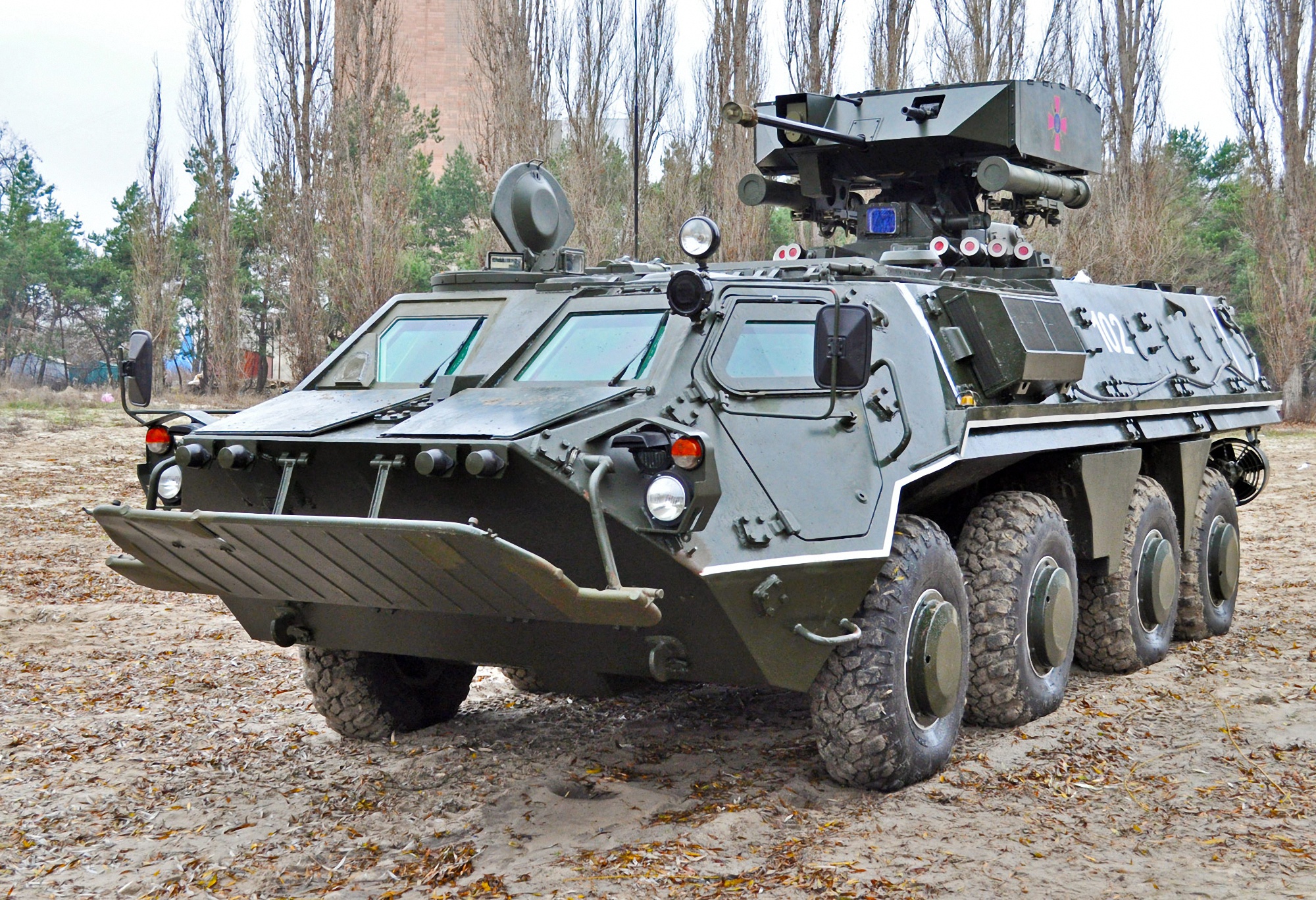A robust military vehicle, specifically an eight-wheeled armored truck, stands prominently in a natural outdoor setting. The sky above is clear, accentuating the contrasting colors of the surrounding trees—some clad in lush green foliage, others barren and brown, signaling the changing seasons. The ground is a mosaic of scattered leaves, twigs, and dirt, adding to the rugged environment.

The vehicle, painted primarily in black, features the identification number "10102" on its side. It is equipped with a formidable turret mounted on top, signifying its combat-ready design. Visible are three windows, although there are likely more, and an array of approximately six headlights ensuring visibility in various conditions. A distinctive, protruding structure at the front of the vehicle suggests enhanced protection, contributing to its imposing appearance.

It is morning, and the nascent light enhances the scene. In the distance, a brick building is partially visible, adding a touch of civilization to this otherwise raw and natural landscape. Notably, a hatch or cover on the vehicle's top appears to be raised, indicating accessibility from above. This detailed setting paints a vivid picture of a morning scene where nature and military technology coexist.